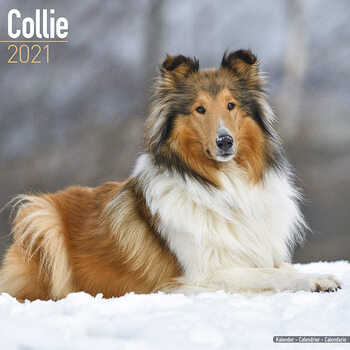This is a detailed image of a Collie dog on the front cover of a 2021 calendar. The Collie, with its brown face accented by darker black fur around its ears and over its eyes, has a white chest, white front paws, and a brown body with lighter blondish highlights near the rear. It is laying down on a pile of snow, looking directly at the camera. The scene suggests a cold, wintery setting with a blurred background where one can faintly make out leafless trees and a grayish sky. In the upper left corner of the image, "Collie" is written in white text, followed by an underscore and "2021" in light brown text. At the bottom left corner, there is a gray rectangle with the word "calendar" written in three different languages.